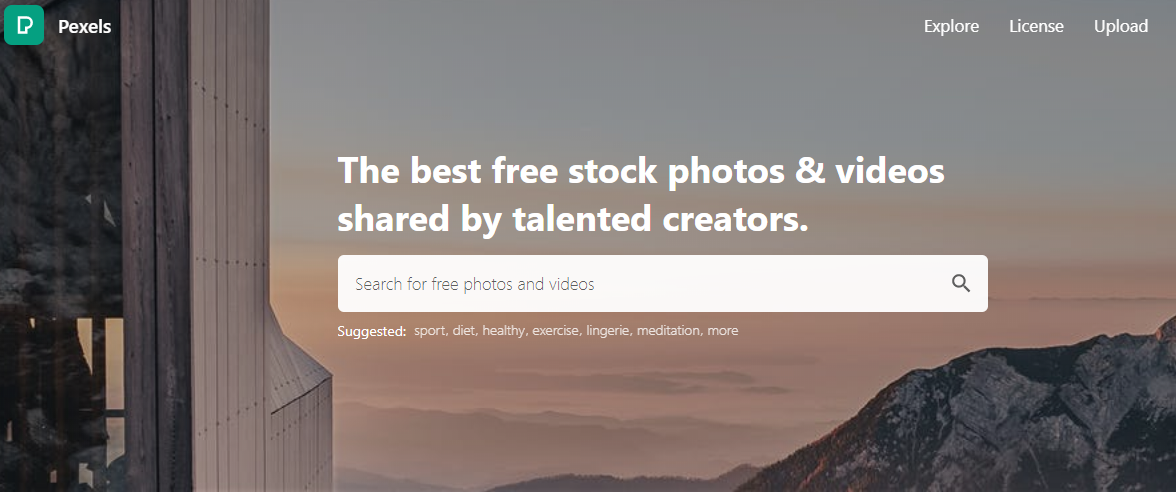The hero image on the website is a wide, expansive screenshot that appears to capture a view from the side of a building, perhaps through a window. The building exterior is made of cement or concrete, and a glimpse of glass is visible on the left side, suggesting the presence of windows. On the right side of the image, the sky is vast, transitioning from a serene blue at the top to a warm pink near the bottom. In the distance, rugged, craggy mountains rise steeply, displaying patches of green and grey. The mountains are bathed in a hazy, pinkish atmosphere that adds to the serene and picturesque quality of the scene.

In the upper right corner of the screenshot, site navigation options are visible, including 'Explore,' 'License,' and 'Upload,' indicating that this is a stock photography platform named Pexels. At the center of the image, text proclaims, "The best free stock photos and videos shared by talented creators." Directly below this statement is a prominent search field inviting users to "Search for free photos and videos." Suggested search terms such as sport, diet, healthy, exercise, lingerie, meditation, and more are listed underneath the search bar. Notably, the webpage lacks additional calls to action such as sign-up buttons or pricing information, focusing solely on encouraging users to begin their search.